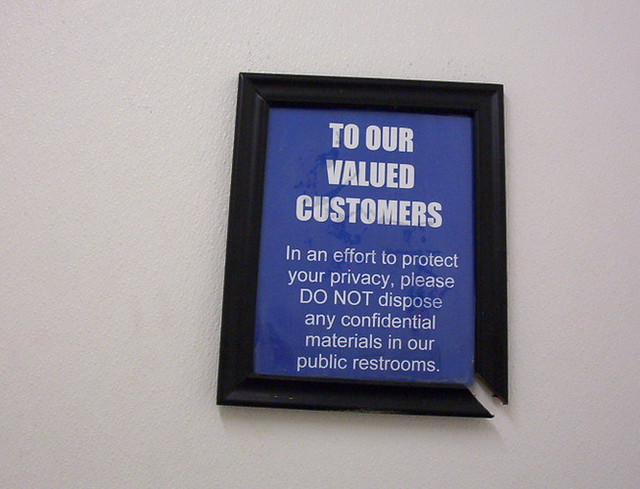In this picture, a framed notice hangs on a cream-colored wall. The black picture frame, which is cracked at the bottom right corner, encloses a sign with a dark blue background. Adorned with white text, the notice begins with a bold headline, "To our valued customers," followed by the message: "In an effort to protect your privacy, please do not dispose any confidential materials in our public restrooms. Thank you." The frame around the notice shows visible wear and tear, including stains and signs of water damage.